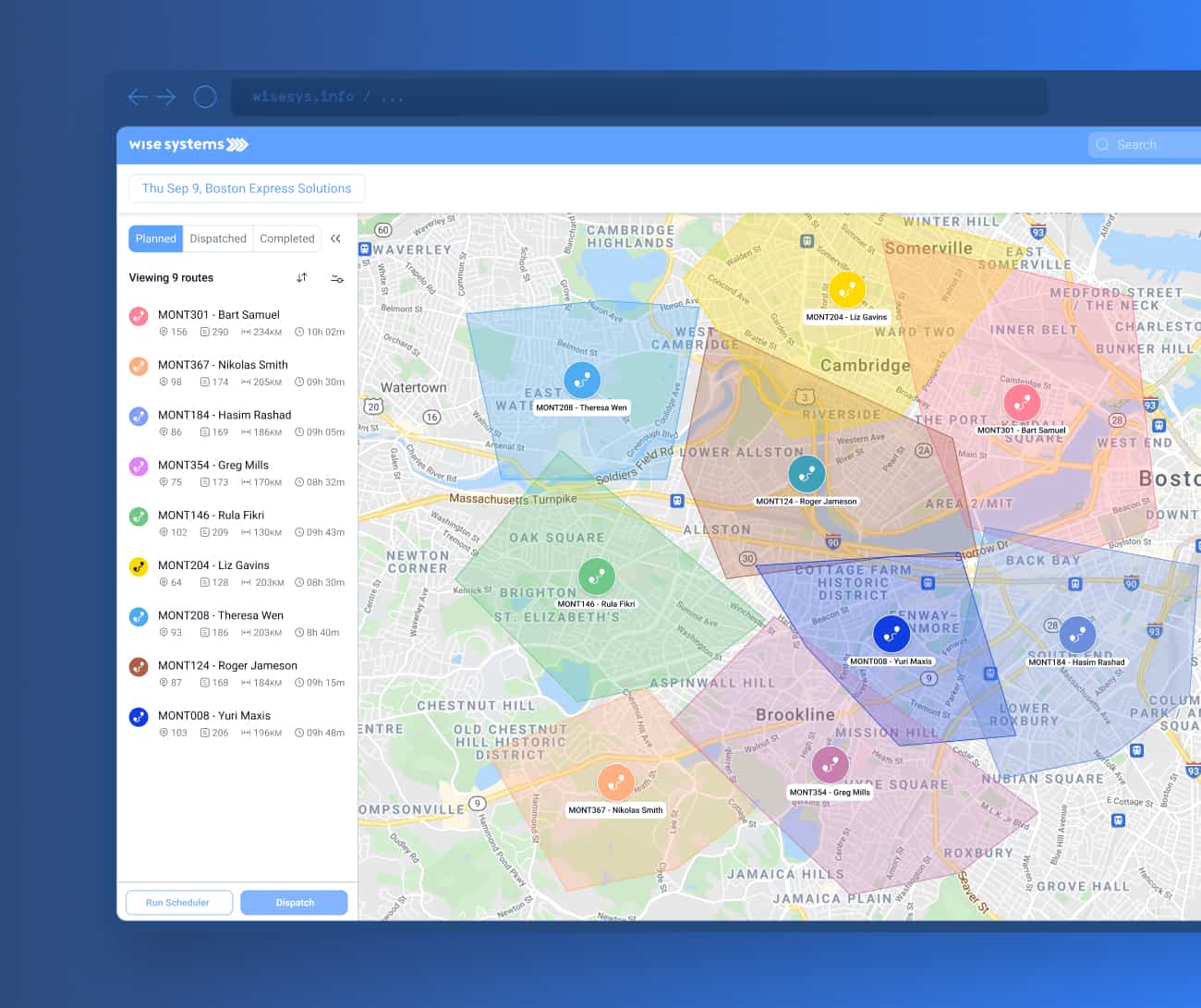The image is a detailed screenshot of a GPS navigation system interface, specifically from WISE Systems. At the top, the WISE Systems logo is prominently displayed in white. Below the logo, three right-pointing arrows are visible. The heading beneath this reads "Thursday, September 9th, Boston Express Solutions."

The interface is divided into three tabs labeled "Planned," "Dispatched," and "Completed." The "Planned" tab is highlighted in blue, indicating that it is currently selected. Under this tab, there is a list of nine planned routes. Each route is labeled with a code starting with "MOTS" followed by a number and the name of the assigned individual:

1. MOTS 301 - Bart Samuel
2. MOTS 367 - Nicholas Smith
3. MOTS 184 - Haseem Rashad
4. MOTS 354 - Greg Mills
5. MOTS 146 - Rula Fikri
6. MOTS 204 - Liz Gavins
7. MOTS 208 - Teresa Nguyen
8. MOTS 124 - Roger Jameson
9. MOTS 008 - Yuri Maxis

To the right of the route list, a map is displayed, showing different colored shapes that correspond to the various routes listed. These shapes are likely used to visually represent the routes on the map, facilitating easier navigation and route management.